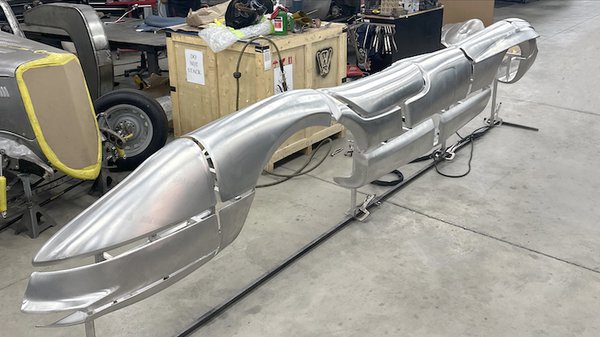This image captures the interior of a workshop or factory environment, showcasing a partially constructed vehicle, possibly an aerodynamic high-speed land vehicle similar to a rocket car. The setting features a large, horizontally aligned, rectangular space with a mix of gray and brown cement slabs on the ground. Dominating the center of the picture is a metallic structure. The object extends from the lower left corner towards the upper right, with its sleek, rounded, and pointed front, indicative of high-speed design for minimized air resistance. Its rear end is also rounded, suggesting an aerodynamic form. 

This metallic piece, with a gray and brown color blend and chrome-like sheen, appears to be the base frame of the vehicle, currently devoid of wheels, a motor, or other components. It resembles a skeletal framework that includes potential wheel wells on both the left and right sides. The item is supported by a series of thin metal black bars or pegs.

In the background, to the upper left, there is a light wooden crate adorned with various objects including a hose hanging from it, indicative of the workshop environment. Nearby, other machinery and vehicles are visible, including a partially discernible vehicle sporting wheels. A toolbox and various instruments are also visible to the left, contributing to the impression that this is a space dedicated to the construction and assembly of high-speed vehicles.